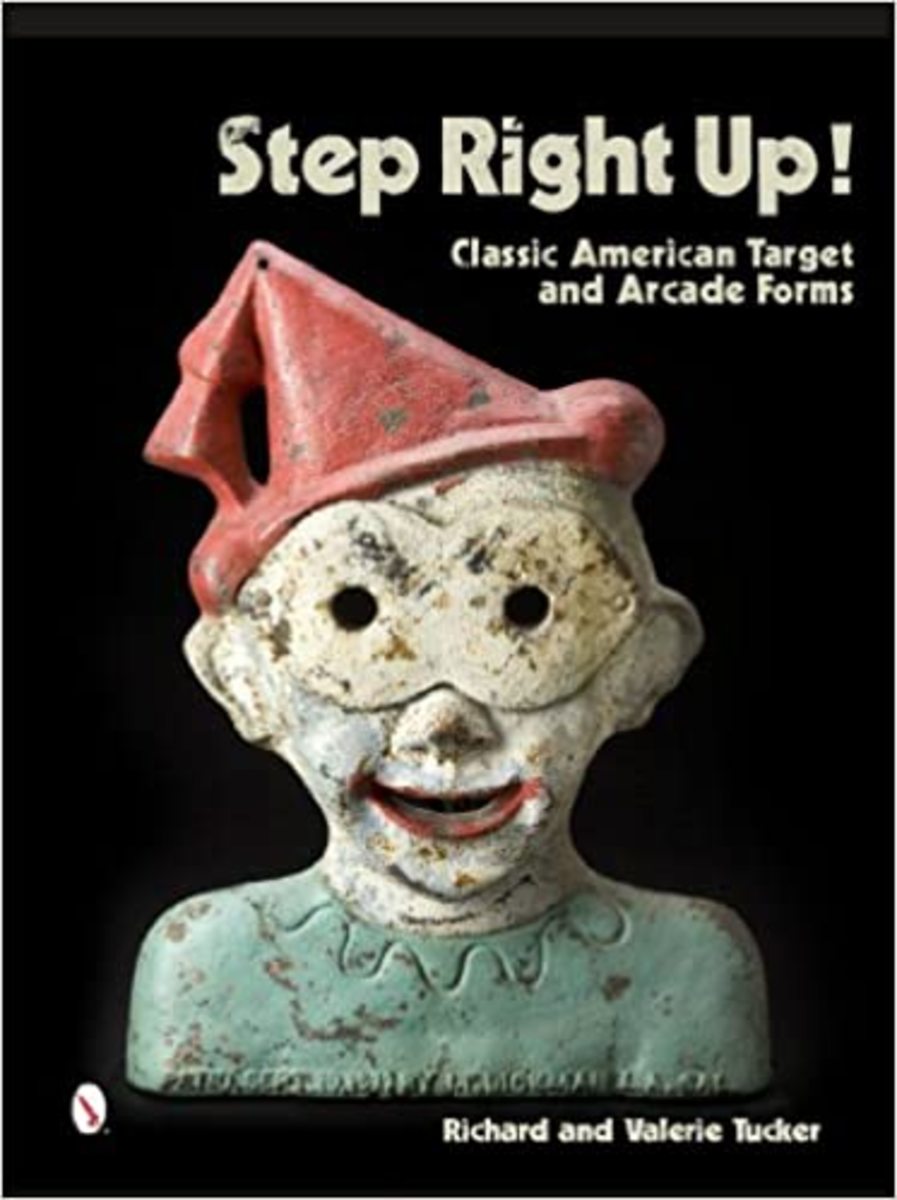The image is the front cover of a book with a solid black background. At the top right, it prominently features the bold white text: "Step Right Up!" with an exclamation point. Below it, in smaller white letters, it says, "Classic American Target and Arcade Forms." The central figure in the image is a painted representation, possibly a figurine or illustration of a clown. The clown has a red, triangular cone-shaped hat with a small tassel hanging from it, slightly askew on its head. Its face is painted white, with white eye covering or goggles in a figure-eight shape, and red painted lips. The clown is wearing a blue upper garment, though the image cuts off below its shoulders, with a visible print mark across its chest. In the bottom right corner of the cover, the names "Richard and Valerie Tucker" are printed. There is also a circle with the letter "J" inside it, located in one of the corners of the cover.